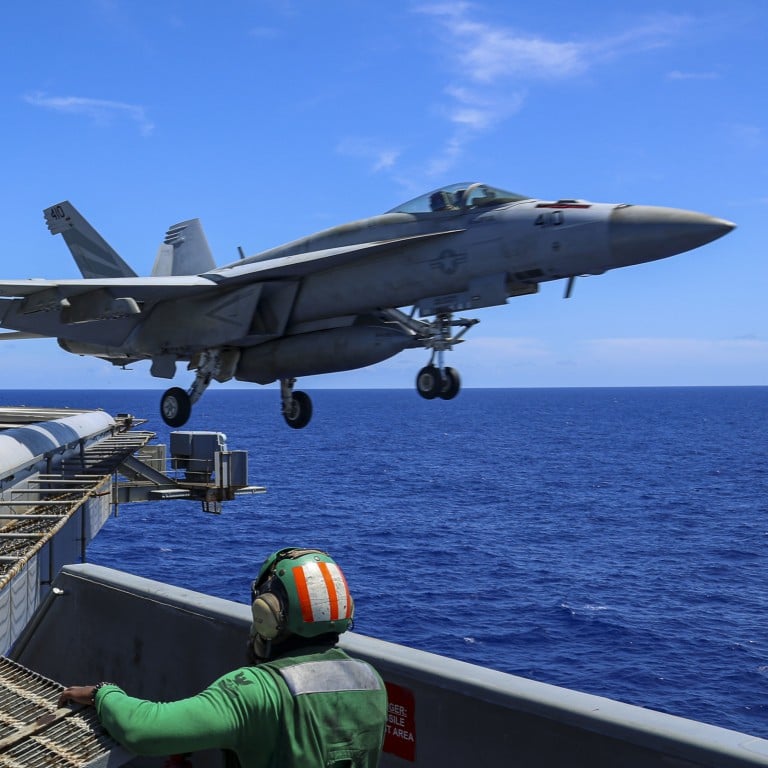The image captures the moment a gray military fighter jet, featuring a sharply pointed nose and a domed cockpit, is taking off from an aircraft carrier in the middle of the ocean. The calm ocean stretches out in the background, meeting a clear blue sky with only a few wispy clouds near the horizon. The jet, which has its landing gear retracted and an underbelly missile visible, dominates the middle of the frame. In the bottom left of the photo, a man stands on the ship's deck, facing away from the camera. He is dressed in a green jumpsuit and helmet, adorned with a white square and red stripes on the back, and wears a headset with protective earwear, indicating the loud environment. The aircraft carrier's deck and a light gray wall are also visible, adding to the maritime setting.